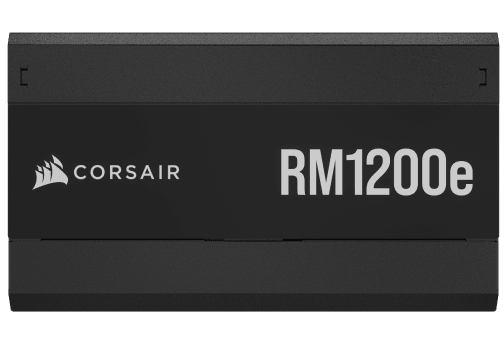The image features an electronic product, likely a rechargeable battery or a similar device, with a high-contrast color scheme. The product has a rectangular shape and seems to be constructed from a black or dark gray plastic. The overall design includes multiple gray and black sections: a thin gray border at the top, a lighter gray section below it, followed by a prominent dark gray border about five times larger, and then a central section nearly three times the size of the last border.

On the left side of the device, there is the Corsair logo, depicted as a series of six white thorn-like or shark fin shapes. Adjacent to the logo, the brand name "CORSAIR" is displayed in large white capital letters. To the right of this branding, the model number "RM-1200E" appears in bold white text, with the "E" in lowercase. This text is considerably larger, likely twice the size of the Corsair logo, making it highly visible.

The device also features some detailing in the form of notches on the upper left and upper right corners, which might suggest it can connect to other components or systems. The background of the image is plain white, further emphasizing the black box and its distinct features like contrasting gold and black bars below the text.